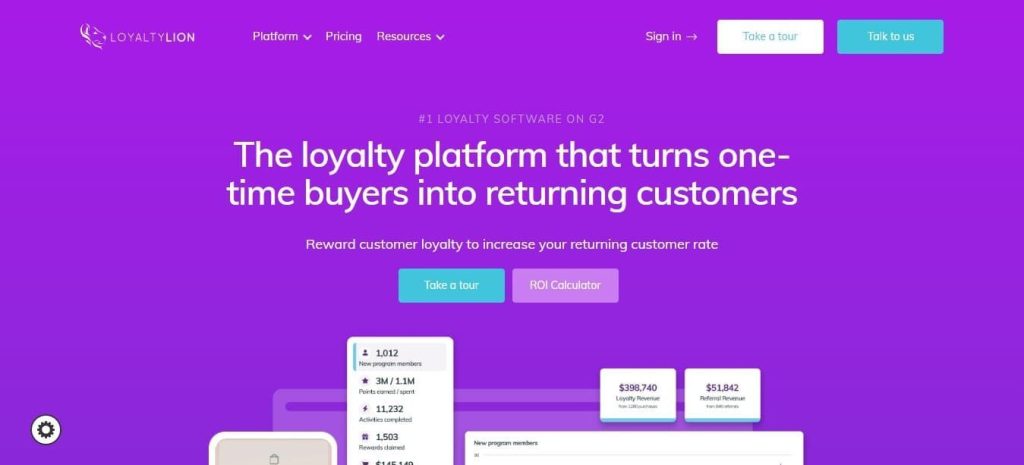The image depicts a webpage dominated by a light violet background. On the top left corner of the page, the logo "Loyalty Lion" is prominently displayed. Adjacent to the logo, the navigation menu items "Platform," "Pricing," and "Resources" are listed in white font, each accompanied by a downward-facing arrow.

On the top right corner, a "Sign In" button directs users to log in, marked by an arrow pointing right. Below it, two buttons stand out: a white button with turquoise font labeled "Take a Tour," and a turquoise button with white font labeled "Talk to Us."

Centrally positioned on the page, an attention-grabbing headline reads, "The number one loyalty software on G2," followed by a detailed description that states, "The loyalty platform that turns one-time buyers into returning customers. Reward customer loyalty to increase your returning customer rate." This text is presented in varying font sizes and styles, all in white.

Below this description, two centered buttons offer further engagement options: a turquoise button with white font that says "Take a Tour," and a light violet button labeled "ROI Calculator."

In the bottom left corner, there is a distinctive icon—a white circle with a black outline containing a sun graphic. At the very bottom of the page, a graphical representation includes what appear to be the tops of phone screens displaying numbers and percentages, suggesting data or stats related to the platform.

Overall, the layout and color scheme are aesthetically unified, combining shades of violet, turquoise, and white to create a visually appealing and functionally clear webpage.